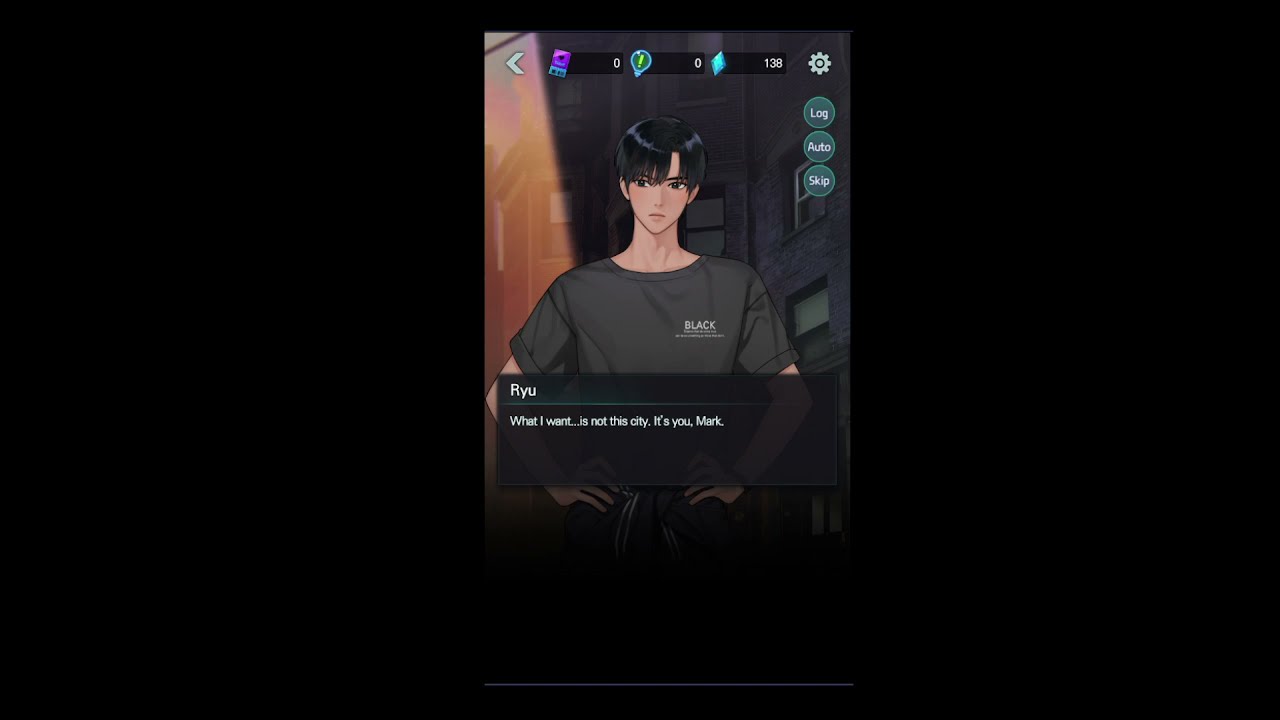The image is a screenshot from a video game, predominantly black with two rectangular black bars on the left and right sides, making the central game image appear vertical and taller than it is wide. At the center is an animated character, an Asian individual named Ryu, identifiable by short, straight black hair that falls to his eyebrows and just touches his ears. Ryu has a narrow chin and fair skin and is wearing a black t-shirt with the word "black" printed in white. In front of him, there's a gray text box displaying his name, "Ryu," and his dialogue: "What I want is not the city, it's you Mark." Above Ryu, game statistics are visible, including a blue diamond with the number 138, a light bulb icon with a green exclamation point, and a purple ticket-like icon. There are also icons on the upper right side of the screen, including settings, log, auto, and skip options.